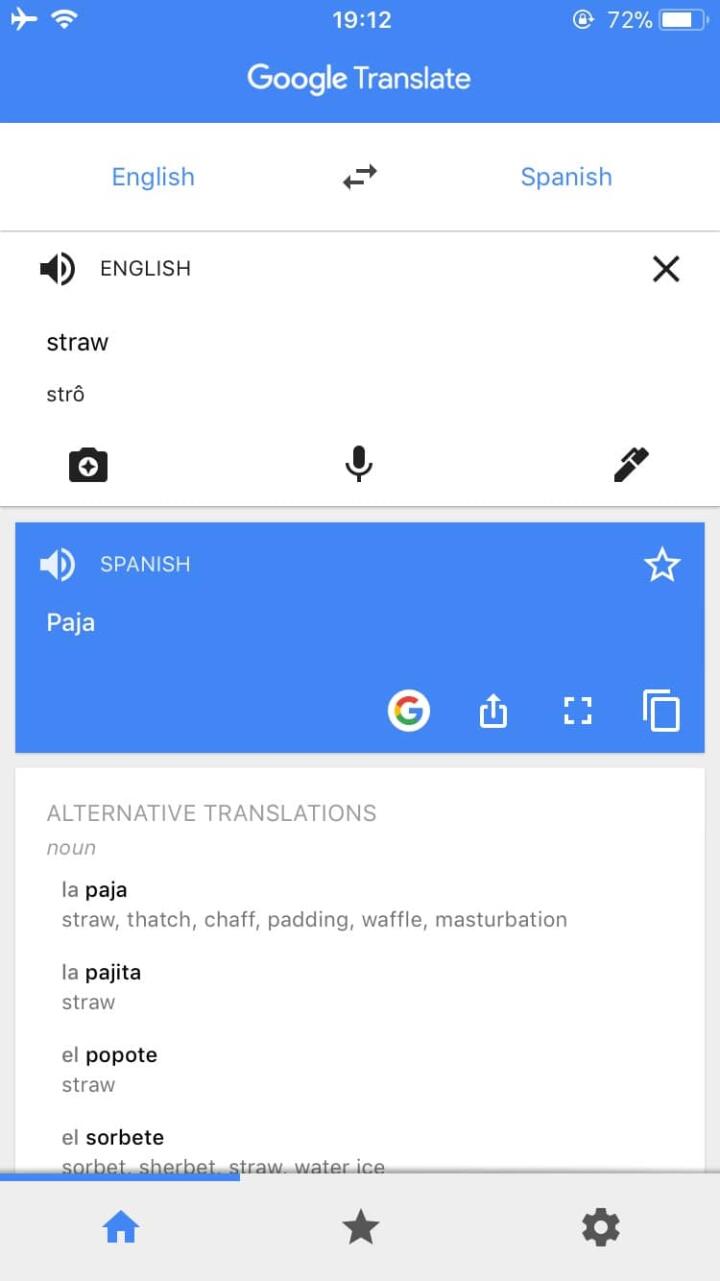The image is a screenshot displayed in portrait mode. The top stripe spans from the upper left to the upper right and is colored blue. 

- **Top Row**:
  - **Left**: Airplane mode icon.
  - **Center**: The time "19:12".
  - **Right**: The battery level at "72%".
  
- **Second Row (still blue)**: Features the Google Translate logo.

- **Third Row (white background)**: 
  - **Left**: "English".
  - **Right**: "Spanish".
  - **Center**: Arrows indicating bidirectional translation.

- **Fourth Row (white background)**: 
  - **Left**: An audio icon labeled "English".
  - **Right**: A black "X" icon.

- **Fifth Row**: 
  - **Text**: The word "straw", followed by its phonetic transcription "S-T-R-O" with a small umlaut over the "O".
  - **Icons**: Suitcase, microphone, and pen.

- **Sixth Row (blue background)**: 
  - **Left**: The word "Spanish" with a sound icon.
  - **Right**: The translated word "paja". An open arrow is also depicted.

- **Underneath**: Features the Google icon, upload, expand, and copy options.

- **Alternative Translations Section**:
  - Lists various translations and meanings:
    - **Noun**:
      - "la paja" – straw, thatch, chaff, paddling, waffle, masturbation.
      - "la pajita" – straw.
      - "el popote" – straw.
      - "el sorbete" – sherbet.

- **Bottom Left Corner**: Displays a blue house icon, next to a black star and black settings icon.